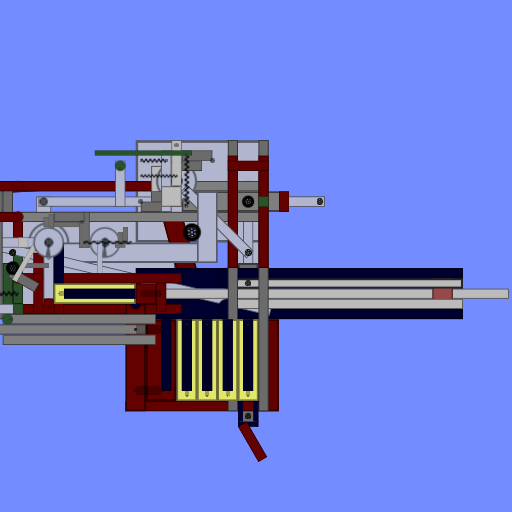Detailed Caption: This image features a computer-rendered schematic of a mechanical apparatus against a light blue background. Dominated by the colors red, yellow, and black, the 2D graphic prominently displays four yellow rectangles with black inner rectangles at the bottom, reminiscent of piano keys. A fifth yellow rectangle with a black inner section is positioned perpendicularly slightly to the left of the main four. Extending to the right from these rectangles is a tube-like structure, capped with a flange, perhaps resembling part of a piston. Additionally, a smaller tube emerges from the top of the apparatus and stretches off to the left, out of the frame. While the schematic may hint at an engine or complex mechanical system, its precise function remains ambiguous, straddling the line between a technical drawing and a form of industrial art.